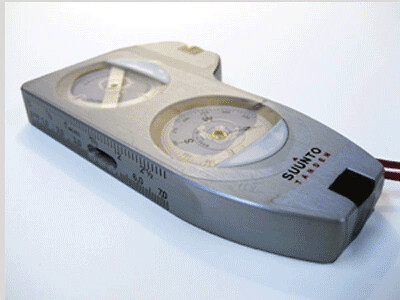The image displays a unique measuring device, which appears to be of an unfamiliar type. The device rests on a stark white tabletop that features a slight shadowed area adding some depth. Constructed from gray metal, the device has a subtle black portion at its base. 

The top layer of the device is inscribed with various texts, while the base prominently displays the brand name "SUUNTO" followed by "TANDEN." The device features two circular dials encased in glass. The lower dial contains a white semicircle and functions as a compass, marked with the cardinal directions: North, South, East, and West, though other details are illegible. The upper dial has another white semicircle towards the right, but lacks discernible markings. Additionally, a ruler with precise hash marks is integrated along the side of the metal body, suggesting its use for detailed measurements.